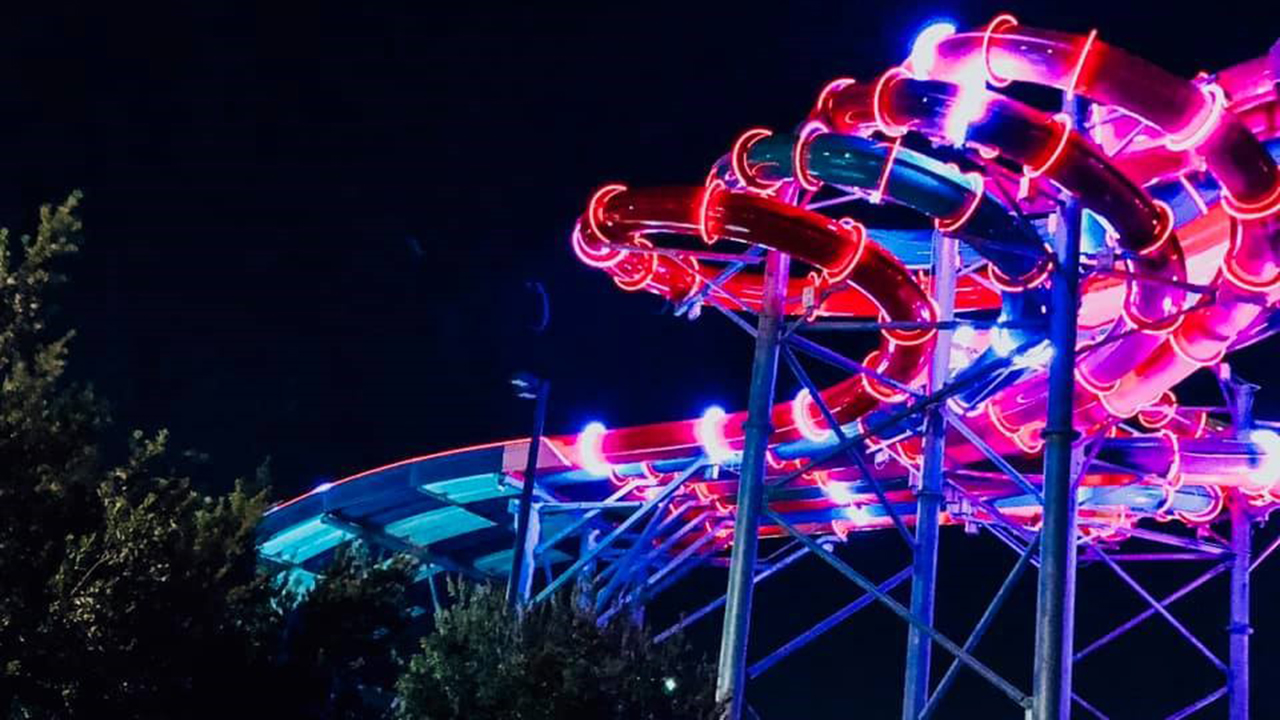In this vibrant nighttime image, an amusement park ride dominates the scene, bathed in neon lights. The central focus is on a twisted array of tubes, most likely part of an elaborate water slide or a similar attraction. The tubes, illuminated with neon red, blue, magenta, and pink lights, spiral and loop before cascading into an open slide section. This intricate structure is supported by a visible scaffolding system, elevated against a backdrop of a night sky tinged in deep blue and black. To the left, large green trees or shrubbery add a natural element to the otherwise mechanical scene. The ride's glowing lights create an enchanting contrast against the dark sky, invoking the lively, festive atmosphere of a carnival or amusement park at night.